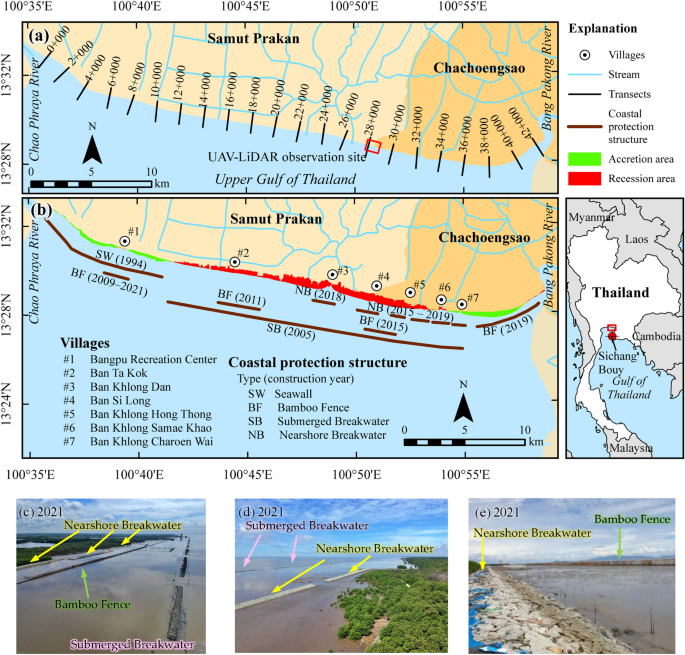This detailed illustration and diagram set focuses on coastal protection structures in the Upper Gulf of Thailand. At the top, two maps provide an overview: the first displays LIDAR observation sites with corresponding numbers, while the second, detailed with a key, indicates the locations of various villages and coastal protection installations such as seawalls, bamboo fences, and breakwaters. An inset pinpoints the exact area within Thailand. Below the maps, three annotated photographs offer a visual complement to the diagrams. From left to right, these photographs depict: an area with a near shore breakwater, bamboo fences extending into the water, and a submerged breakwater farther out; a coastline labeled "D-2021" featuring both near shore and submerged breakwaters; and a third area marked "E-2021" showing a near shore breakwater amidst rocky shoreline and a distant bamboo fence. This composite image thus intricately combines schematic maps and real-world photos to illustrate both the geographical context and physical structures used for coastal protection in this part of Thailand.